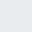A light gray, digital square, approximately two inches by two inches, is displayed on a clean, white background. The square's borders meet precisely at 90-degree angles in all four corners, creating a simple, geometric shape. Its faint gray hue stands out subtly against the stark white backdrop, emphasizing its minimalist design. The image is devoid of any additional elements such as text, figures, or scenery, focusing solely on the unadorned gray square.